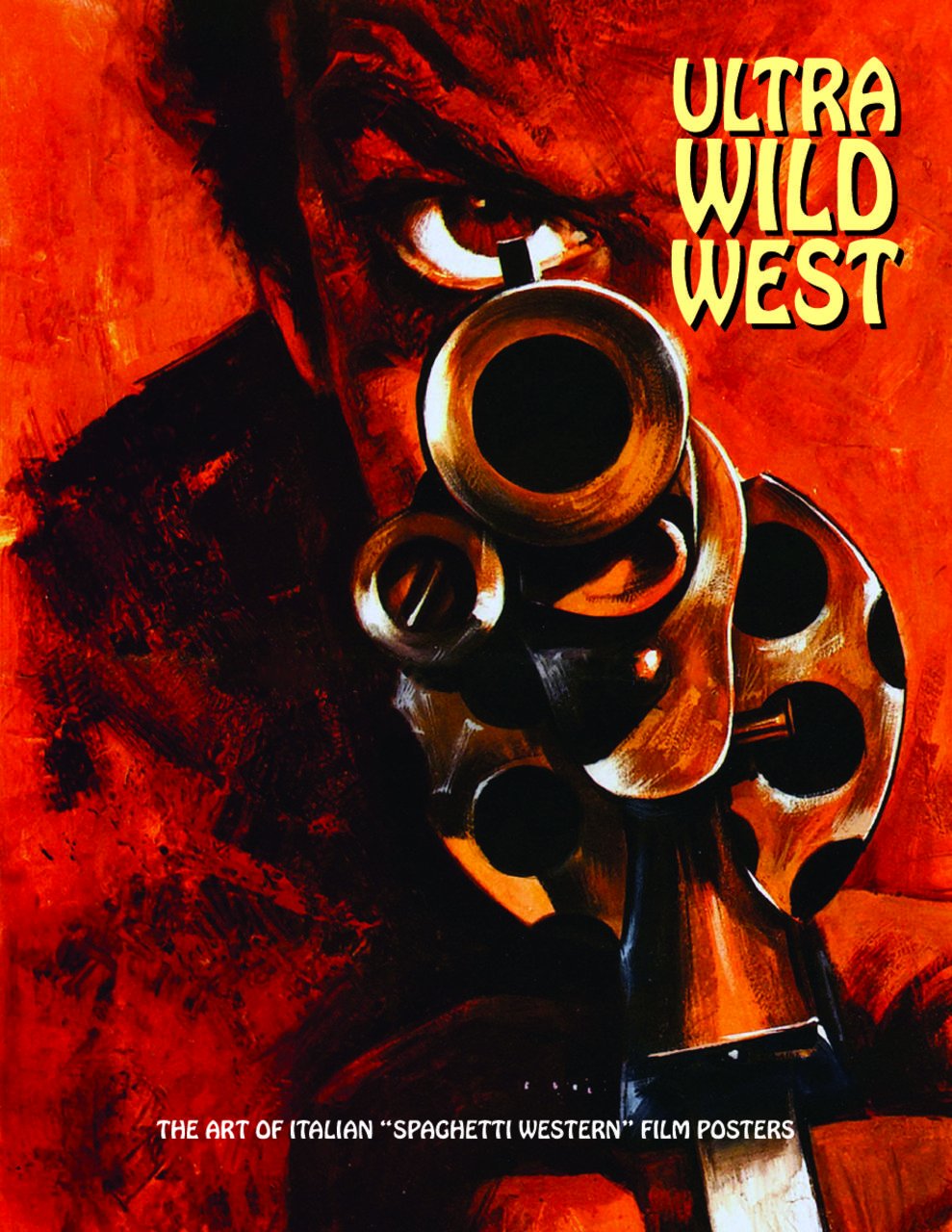The poster for "Ultra Wild West: The Art of Italian Spaghetti Western Film Posters" is a vibrant, stylized depiction set against a bright red, gritty, and grainy background, reminiscent of a charcoal or pastel painting. Dominating the image is the striking close-up of a man's face, only the left half of which is visible, the other half blending seamlessly into the red backdrop. His eye, with its bright white sclera, red iris, and black pupil, is sharply focused down the sights of a shiny silver revolver, pointing directly at the viewer. The man's large coat and frizzy hair contribute to his intense, disheveled appearance. The title "Ultra Wild West" appears in a jaunty, old 70's style yellow font on the right-hand side, while the subtitle "The Art of Italian 'Spaghetti Western' Film Posters" is placed in smaller white text towards the bottom.